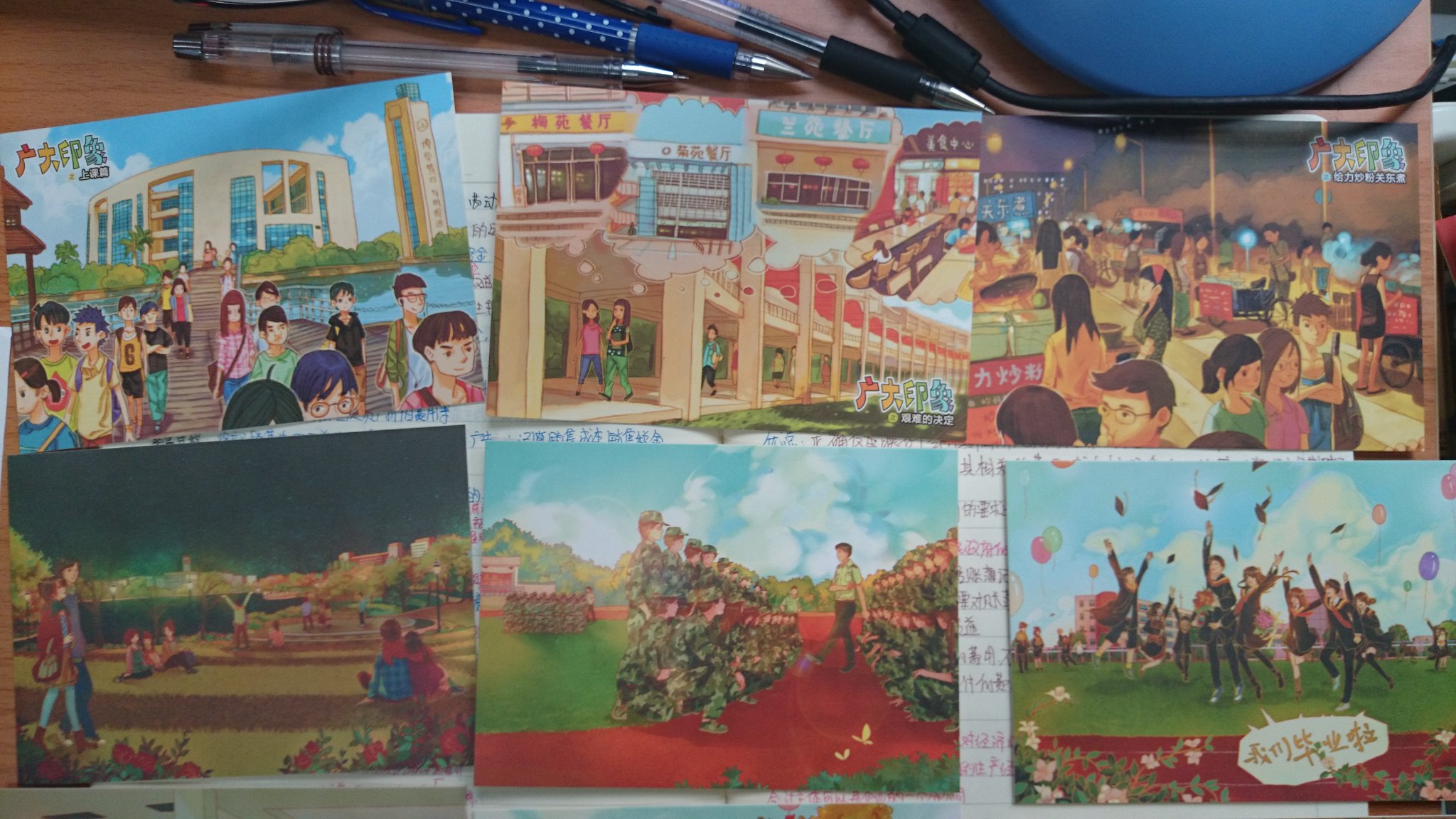This image captures six colorfully illustrated greeting cards or postcards, possibly of Japanese or Chinese origin, laid out on a wooden desk. Each card features groups of young people engaged in various activities. In the top left, there is a circular yellow school surrounded by trees, with children walking out from it. Beside it, the top middle card depicts a scene resembling an outdoor station or open corridor, where children are under an overhead structure, with bubbles indicating their imagination. To the right, the top right card shows an outdoor market or street scene with vendors and customers, set against a nighttime sky. The bottom left card features people walking through another night-time outdoor landscape with some vendors in the background. The bottom middle illustrates people in camouflage uniforms, likely an army, standing in formation on a red road, focused on a central figure. Lastly, the bottom right card portrays a graduation scene where students in black robes are joyously throwing their caps into the air. The setting includes three pens and bits of a blue lamp with a black cord further adding context to the desk environment.